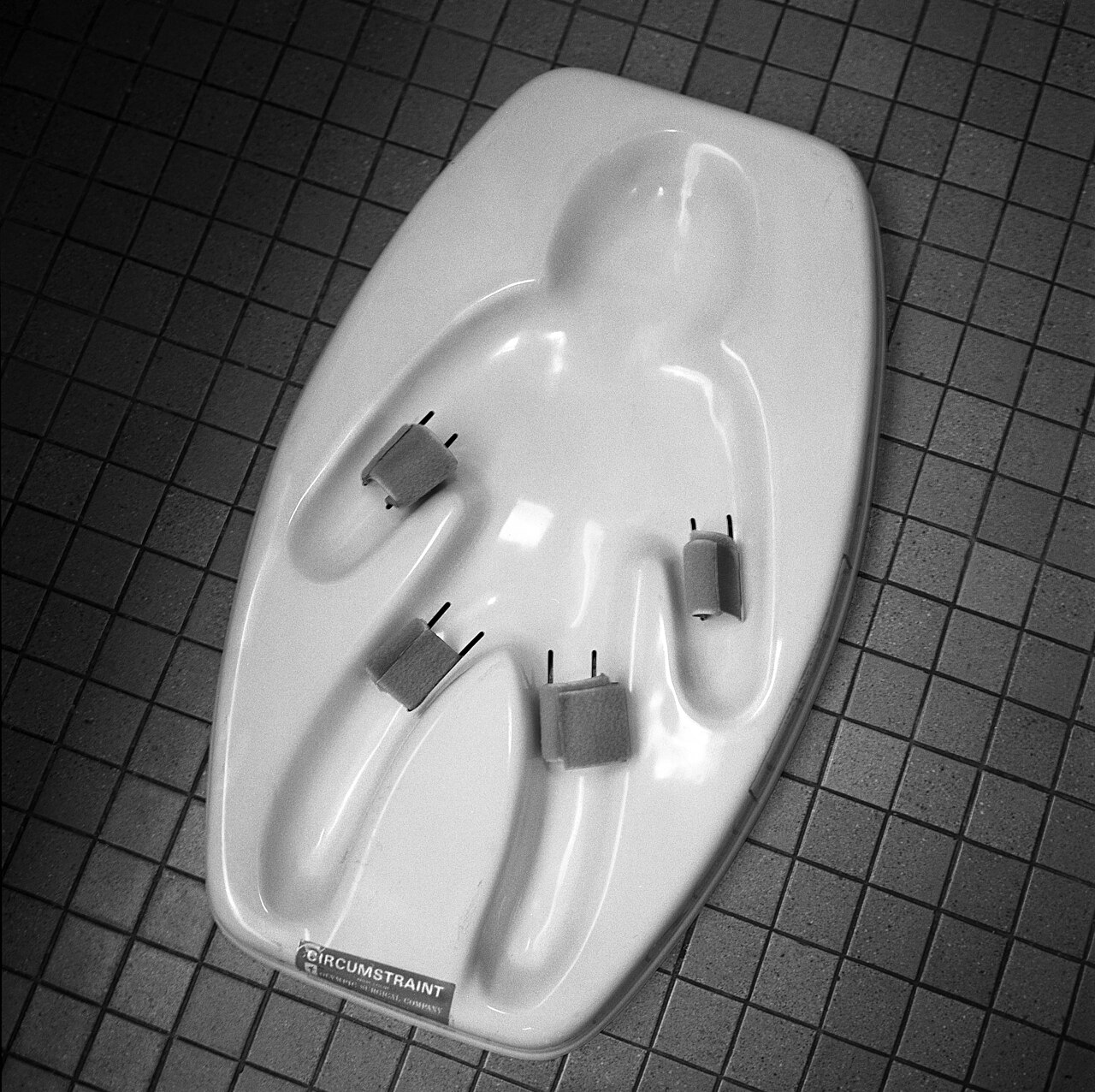The square color photograph features an unusual white plastic tray, resembling a mold, shaped like a doll or small child. Centrally positioned and slightly tilted to the right, the tray has defined indentations for the arms, legs, and head. It rests on a gridded floor or countertop. At the bottom, between the feet, a gray label or sticker reads "Circumstrate." The tray may serve as a restraining system for a small object or figurine, though its exact purpose is unclear. Four round Velcro-like circles, each with two metal prongs protruding, are positioned around the wrist and thigh areas, hinting at a mechanism for securing something in place. The absence of other objects in the frame makes it difficult to gauge the tray's scale.